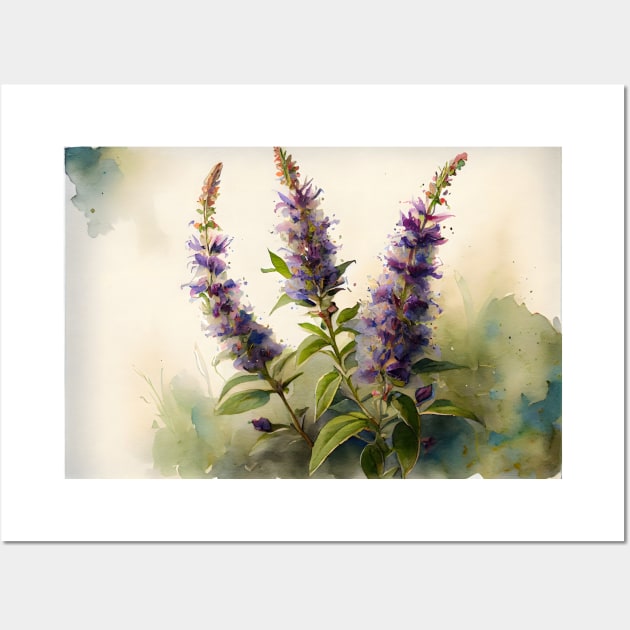This image captures a detailed watercolor painting of a hyacinth plant, digitally rendered and showcased on a white wall with a white border. The focal point of the artwork is three tall, green-stemmed hyacinths adorned with lush green leaves. The flowers bloom in a vivid purple with some scattered purple paint splatters highlighting the delicate petals. The topmost parts of the flowers taper into conical shapes with green seeded portions flecked with red. Surrounding the flowers, the background is predominantly tan, but in the bottom right corner, there is a greenish-gray area enriched with green watercolor blobs to create the illusion of foliage. The flowers emanate upward from the bottom of the image; two stems rise straight while one slightly bends to the left. This painting appears to be professionally presented, as if photographed for an art sale.